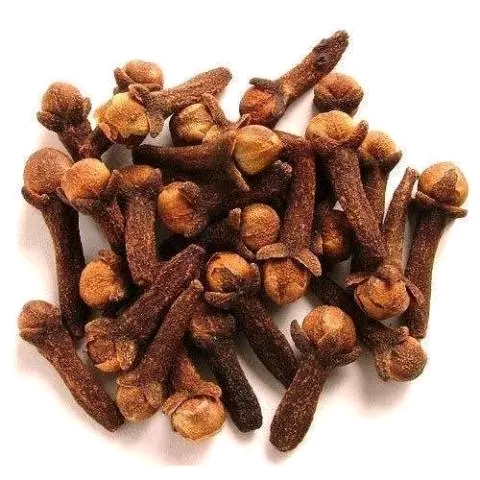The image features a pile of clove buds against a pure white background, creating a stark contrast that highlights their details. The cloves are small, about the size of a small finger, and they are uniformly brown with a distinct color contrast between the parts. Each clove has a dark brown vertical stem that tapers into a lighter brown, round top, reminiscent of a small orb or bud. Some cloves appear very round, while others have a slightly pointy top, suggesting they could open further. The cloves are arranged haphazardly, with some facing up, others down, and a few lying sideways. A closer look reveals that they possess a distinctive texture, with a fuzzy appearance and tiny, curved projections around the top, almost as if holding the orb in place. Scattered among the cloves are small white dots, akin to salt crystals, adding a final layer of detail to the image.